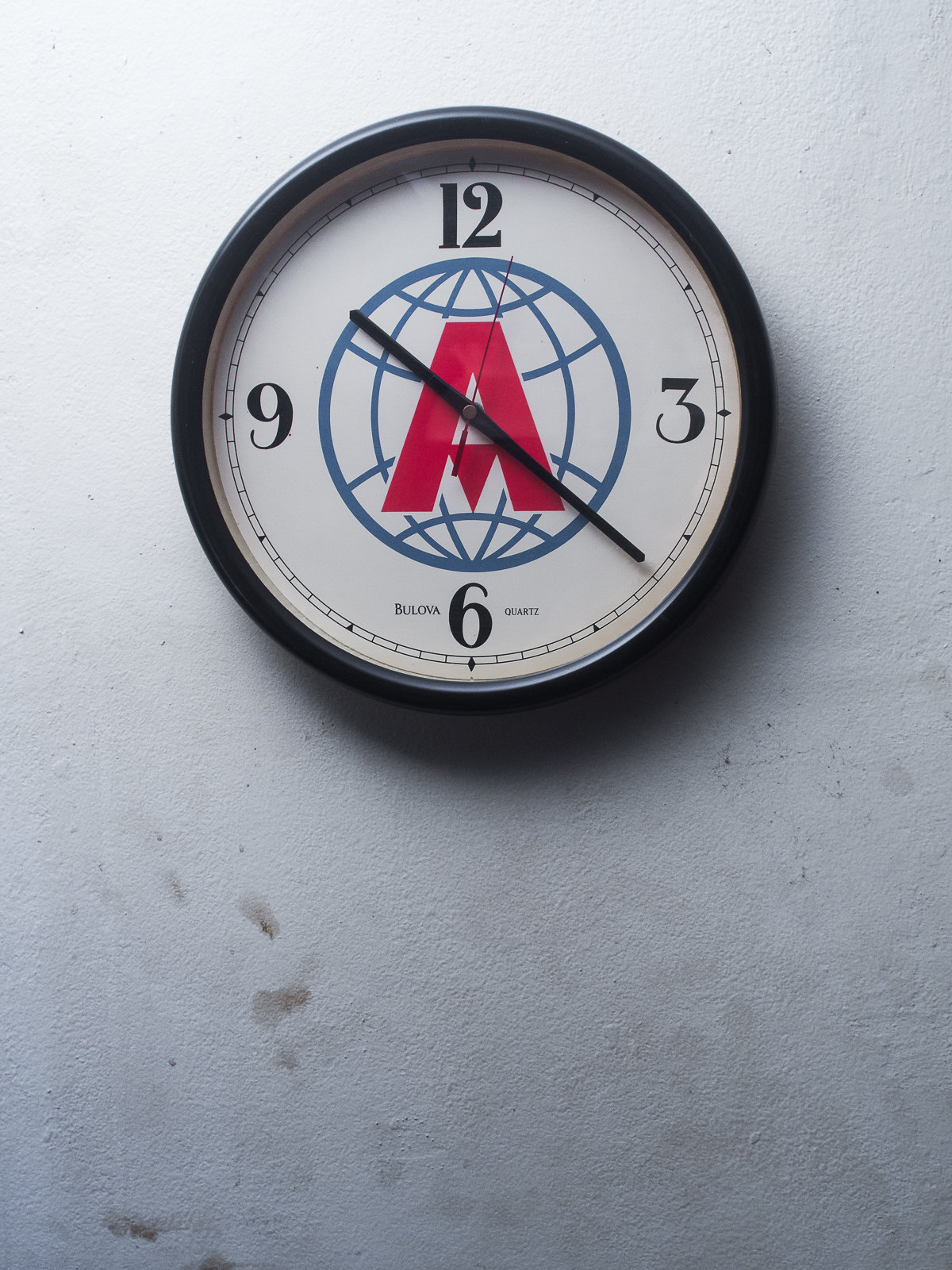The image features a solitary clock mounted on a weathered wall, marred by noticeable black smudges that resemble oily residue. Positioned slightly above the center of the frame, the clock displays the numerals 12, 3, 6, and 9, with small tick marks indicating the remaining hours. Some of these marks are accentuated with darker ridges. The clock's face is adorned with a stylized 'A,' where the crossbar is replaced by an upside-down triangle, set against a backdrop resembling a globe.